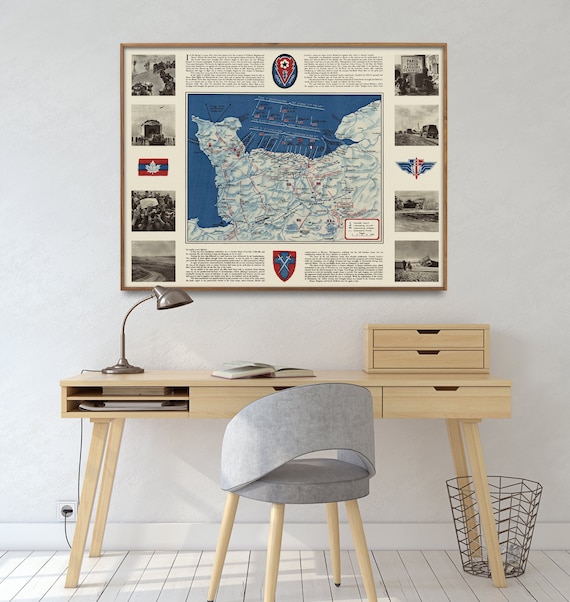The image depicts a Scandinavian-style home office featuring a light beige-colored wooden desk and a modern gray chair with a rounded seat and wooden legs. The desk has two spaces for organization: a set of drawers on the left, a single drawer in the middle, and another narrower drawer on the right. Additionally, there are two box drawers that sit atop the desk. The desk holds an open book in the center and a gray lamp with a visible cord plugged into an outlet. Beneath the desk, a dark gray wire wastebasket is placed, empty. The room's floor is made of light cream-colored wooden slats. On the back wall, a large framed map is displayed with some illegible text and various emblems, including a red shield with a blue cross, an oval shield with blue and red, and a rectangular flag with red and blue stripes and a white maple leaf. The space is complemented by scattered photos around the map, completing the minimalist and functional decor.